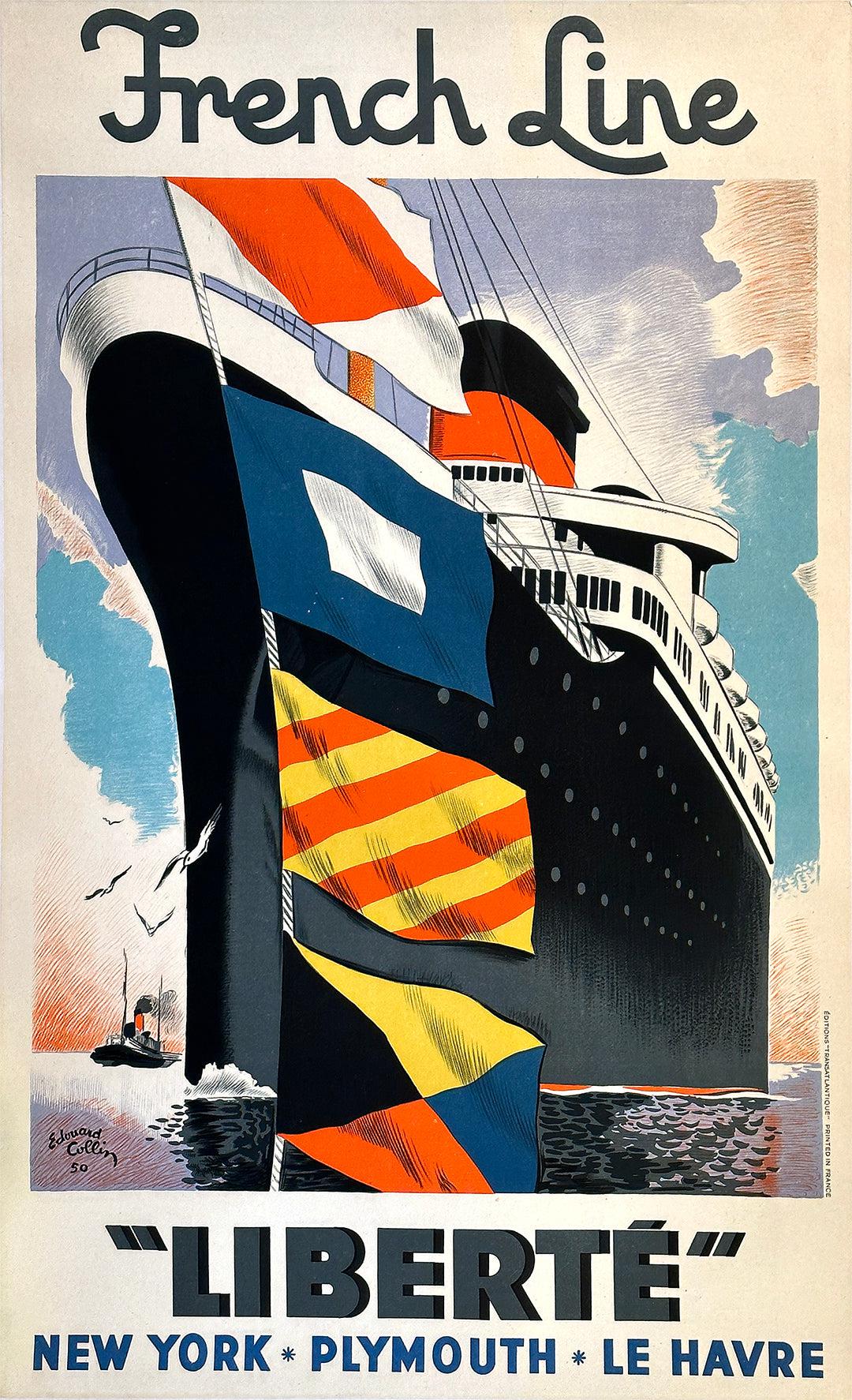This image is a detailed artwork or possibly a vintage advertisement poster depicting an old-fashioned ship. The art is presented within a long vertical rectangular format. At the top, in elegant black cursive font, the text reads "French Line." Below this title, there is a large painted rendition of a ship viewed from the front. The ship's body is predominantly black with a white upper trim, and it features a distinctive black and orange smokestack. A row of four vertically aligned flags is positioned in front of the smokestack, with designs including a white flag with an orange triangle, a blue flag with a white square, and other multicolored flags.

The background of the artwork showcases a vibrant sky filled with purple swirls, complemented by hints of blue, white, and yellow, giving it an almost surreal appearance. The whole composition is set against a medium-shaded tan backdrop. At the bottom of the artwork, the word "Liberté" is prominently displayed in large gray letters enclosed in quotations, followed by the names of cities: New York, Plymouth, and Le Havre, in blue letters. The detailed and colorful nature of the depiction suggests both the grandeur of the ship and the international destinations it connects.